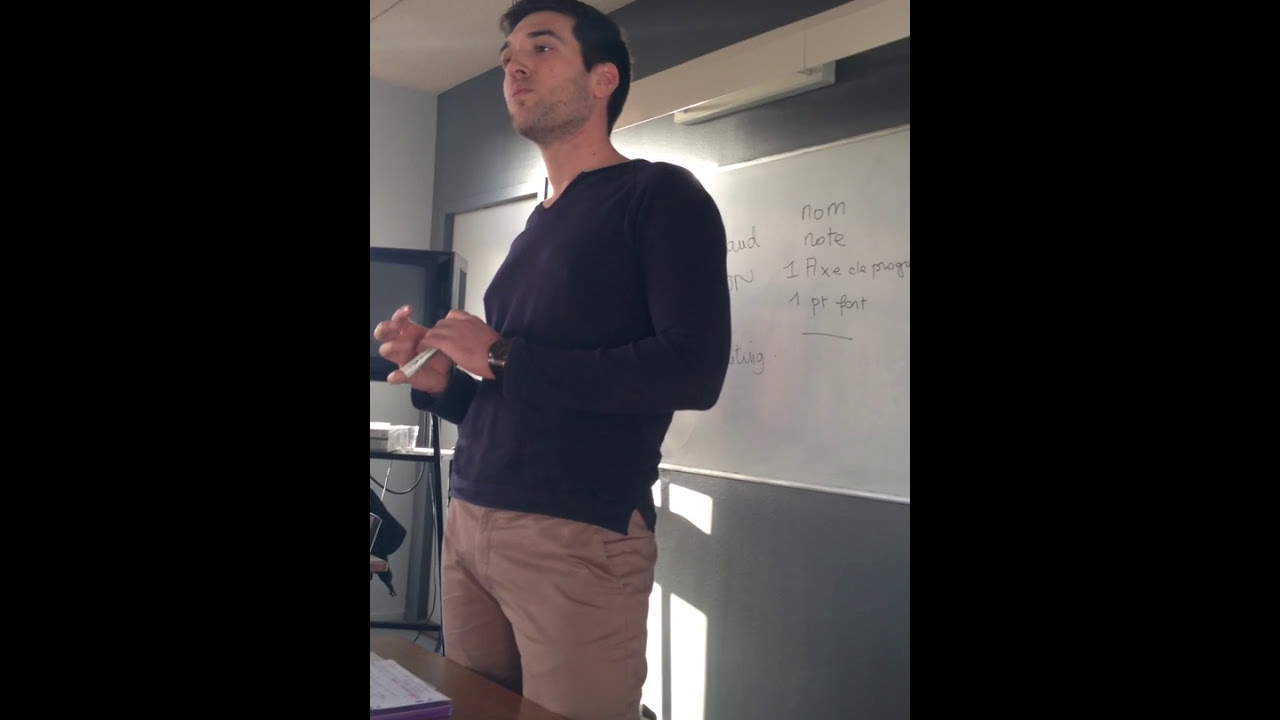In the image, a young man is standing in a classroom or office setting, framed by black borders on the left and right sides, which take up about half of the picture's width. He is positioned slightly to the left in the shot, wearing a long-sleeved black or navy blue shirt and tan khaki pants. The man has short black hair and thin black stubble. He is holding a white dry erase marker in his left hand, with his elbows bent, as if he is giving a lesson or presentation. 

Behind him is a large whiteboard featuring various notes written in black marker, including partially legible text like "nom," "note," "one fix," "one point font," "Nate," "one flex," and "one PT." The whiteboard is attached to a dark gray or greenish wall. To the left of the man, there is a black cart holding an old CRT television, with a cord visibly extending from it. A desk is in front of him, with a piece of paper lying on top. Additional light is streaming from a window, illuminating the area.